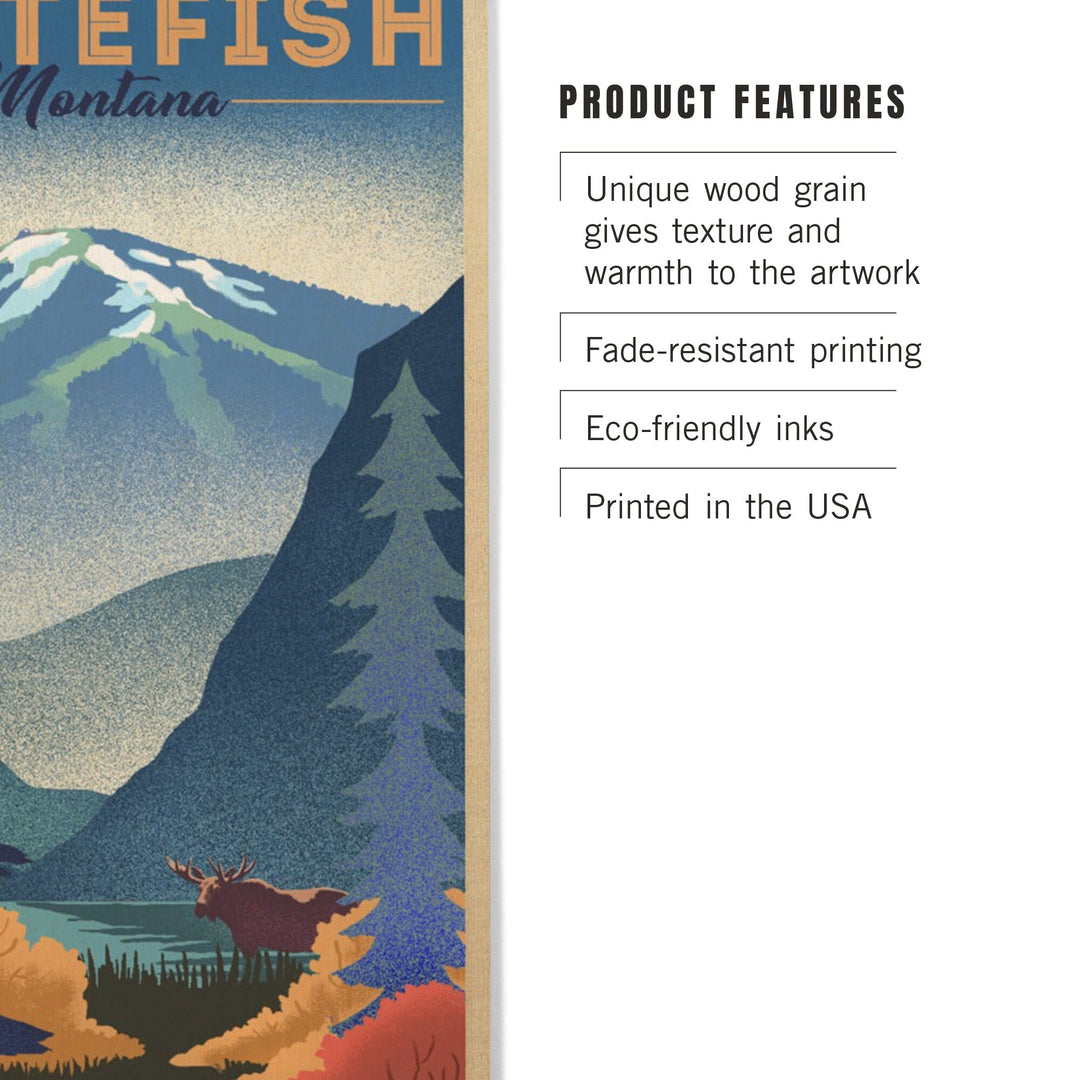The image showcases a section of a nature-themed poster that has been partly cut off at the top and left edges. At the top, there are partial words with "fish" in gold block letters and "Montana" in dark blue or black cursive lettering. Below this, the scene transitions into a beautiful, tall mountain range with snow-capped peaks and green ski trails. Smaller mountains and hills cascade down from the main peaks. On the right-hand side, there is a darker, almost black mountainous range. Nestled within this landscape is a lake, with a large brown moose standing by the water's edge surrounded by tall green grasses and yellow and orange bushes in the foreground. An evergreen tree stands prominently, adding depth to the composition. Additional text accompanying the image highlights the product features of the poster: unique wood grain texture, fade-resistant printing, eco-friendly inks, and proudly printed in the USA. This richly detailed scene appears to be from an advertisement for a print or poster-making service.